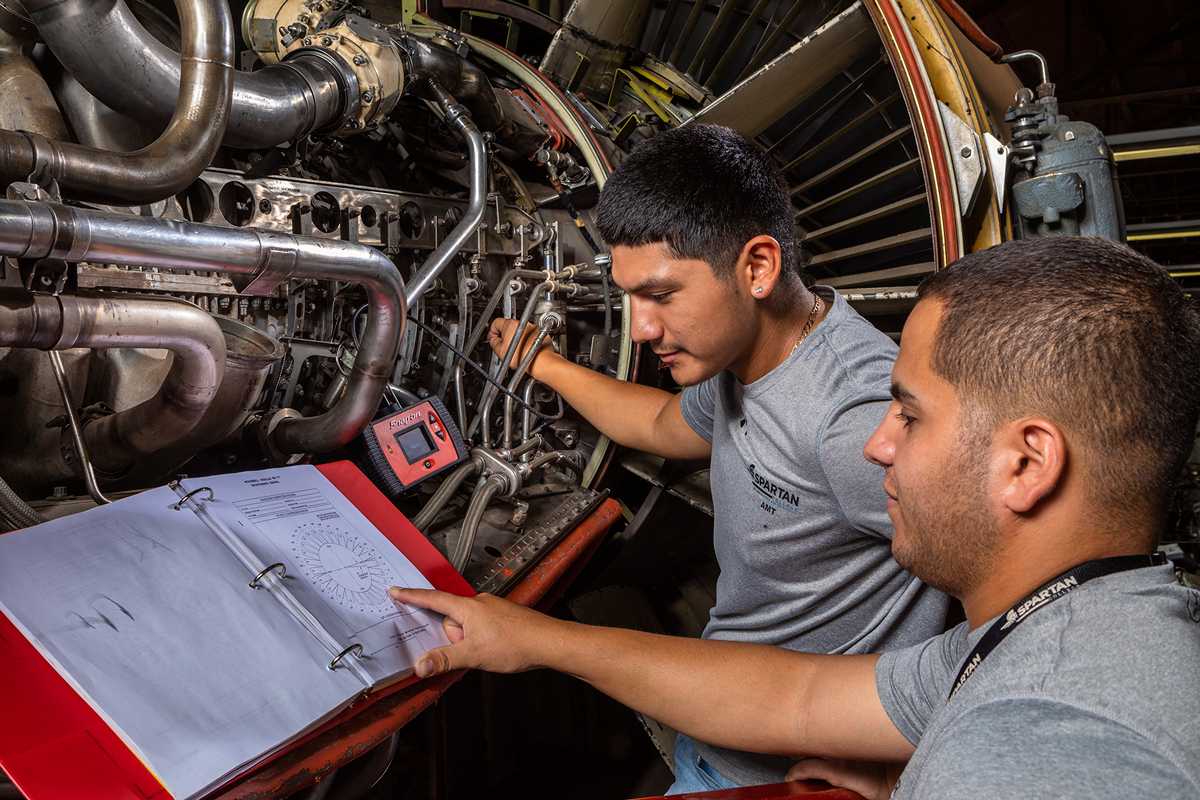In the photograph, two men with brown hair and brown skin are intently working on a large engine decorated with the name "Spartan." Both are dressed in gray shirts. The engine, featuring a prominent fan and an array of metal pipes, wires, valves, and switches, occupies the background and upper left-hand corner of the image. One man is inserting his hand into the engine's components while the other points to a detailed diagram within a white-paged binder that is encased in a red cover. The man pointing to the booklet also wears a black necklace inscribed with "Spartan." An additional device, likely a diagnostic tool, is visible leaning against the engine. Both men appear to be focused and engaged with the task at hand, illustrating their focus on the detailed mechanical work.